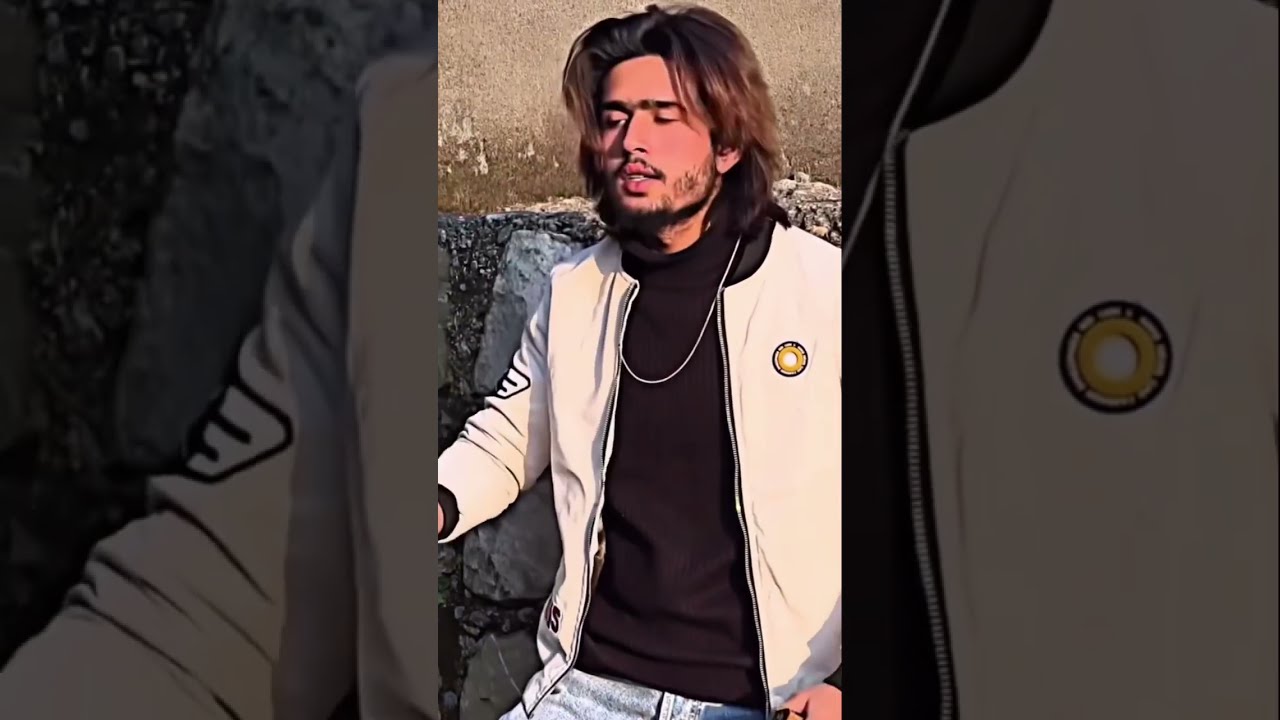The image features a man with long, stringy, brown hair, a scraggly beard, and heavy eyebrows, looking slightly to the lower left. He is dressed in a white jacket adorned with an emblem outlined in blue with a yellow or green center on its right side, over a black turtleneck, and is wearing blue jeans, partially visible. A gold chain is around his neck. His face appears red, possibly due to photo saturation. The background consists of a textured cement wall with rocks and bricks, shifting in color from black and gray to brown near his lips. The photo is a three-panel composition: the left panel shows a close-up of the man's right sleeve while the right panel highlights his left shoulder. The central panel gives a full view of the man. The side panels are essentially enlarged, grayscale fragments of the main image, creating a subtle border effect. Uniquely, a segment of the image includes the inside of a gray jacket, from which the photograph of the man seems to be emerging.